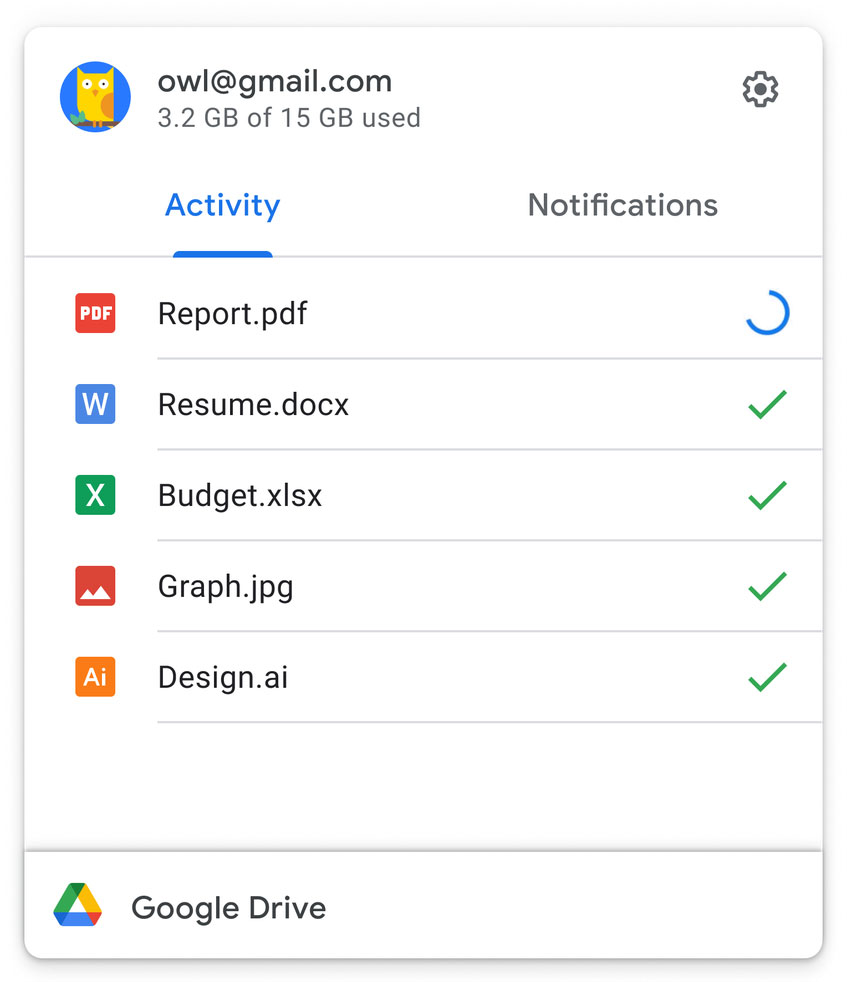This screenshot provides a detailed view of a Google Drive interface. At the top of the screen, the profile picture is an illustrated yellow owl, and next to it, the email address "owl@gmail.com" is displayed. Below this, storage usage is indicated: "3.2 GB of 15 GB used." Two tab options are visible: "Activity," which is highlighted in blue, and "Notifications."

In the upper right corner, there is a gear icon, signifying settings. Under the "Activity" tab, there are five distinct activity items separated by light dividers:

1. **Report.pdf** - Icon: Red square with white "PDF" lettering; Status: A partially filled blue circle indicating it's still loading.
2. **Resume.docx** - Icon: Blue square with a white "W"; Status: Green checkmark indicating successful upload.
3. **Budget.xlsx** - Icon: Green square with a white "X"; Status: Green checkmark indicating successful upload.
4. **Graph.jpg** - Icon: Red square with two white mountains; Status: Green checkmark indicating successful upload.
5. **Design.ai** - Icon: Orange square with white "AI" lettering; Status: Green checkmark indicating successful upload.

At the bottom, the Google Drive logo is displayed to the left of the text "Google Drive."